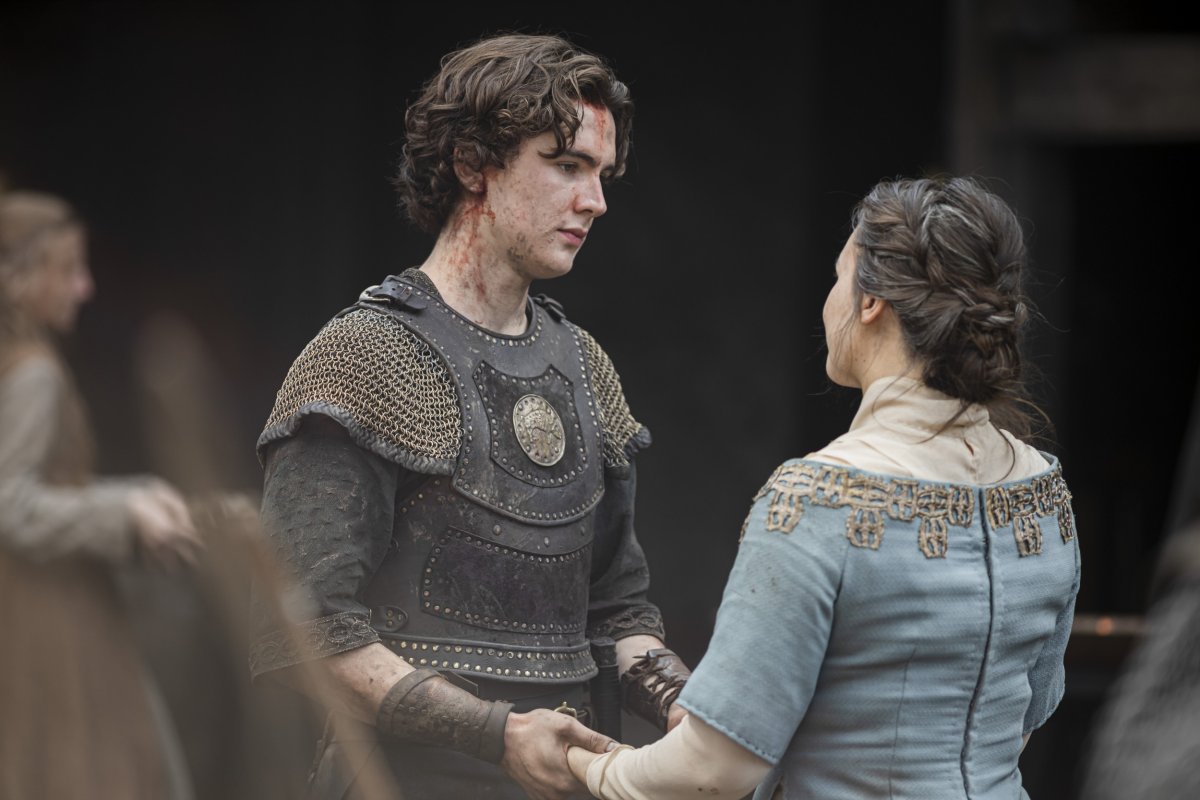The image portrays a scene reminiscent of a historical or fantasy film, featuring a man and a woman holding each other's hands while gazing into each other's eyes. The man, positioned on the left, is adorned in chain mail and brown leather armor with metal embellishments. He has long, curly brown hair and blood streaks on his forehead and beneath his right ear, suggesting he's wounded, possibly from a recent battle. The woman, standing on the right, is dressed in a light blue top over a cream-colored shirt that covers her neck and extends to her wrists. Her gray hair is swept into a braid that falls into a messy bun. The setting exudes an olden times ambiance, reinforced by the armor and the woman's attire. The background is hazy, suggesting a dramatic post-battle atmosphere, with a faint image of another woman walking by in the left corner. This intricate scene captures a poignant moment, perhaps a farewell or reunion, enhanced by the medieval-like costumes and somber expressions.